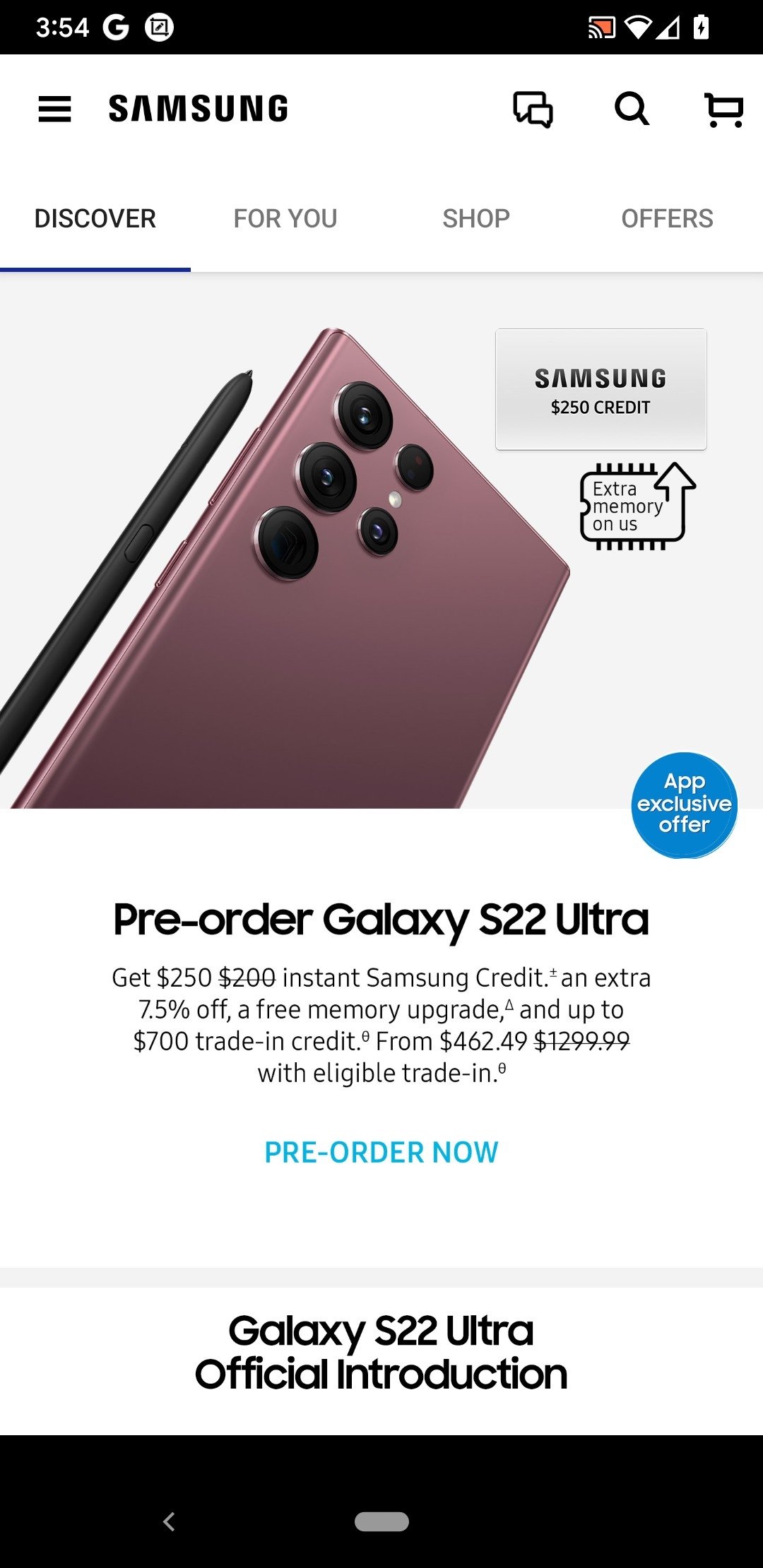A detailed screenshot from a smartphone displays various interface elements and information about a special promotional offer for the Samsung Galaxy S22 Ultra. At the top of the screen, a black notification banner shows the current time (3:54) on the left and a letter "G" on the far right. The battery icon indicates it is almost fully charged. Below, the text "Samsung" appears, accompanied by a search button and a shopping cart icon on the right.

Four tabs lie beneath this header: Discover, For You, Shop, and Offers, with the "Discover" tab currently selected. The main content area displays an image of a phone slightly tilted to showcase its back, featuring multiple cameras. To the left of the phone is a black stylus pen. The phone itself sports a purplish-pink color. In the top right corner of this image, a label reads "Samsung $250 credit," with an arrow and text saying "Extra Memory on Us." Additionally, a blue circle in the bottom right corner of the image states "App Exclusive Offer."

Further details are listed below the image, inviting users to "Pre-Order Galaxy S22 Ultra." The offer includes $250 instant Samsung credit, an additional 7.5% discount, a free memory upgrade, and up to $700 trade-in credit, starting from $462.49 with eligible trade-in. A prominent "Pre-Order Now" call-to-action is provided, followed by the caption "Galaxy S22 Ultra Official Introduction."